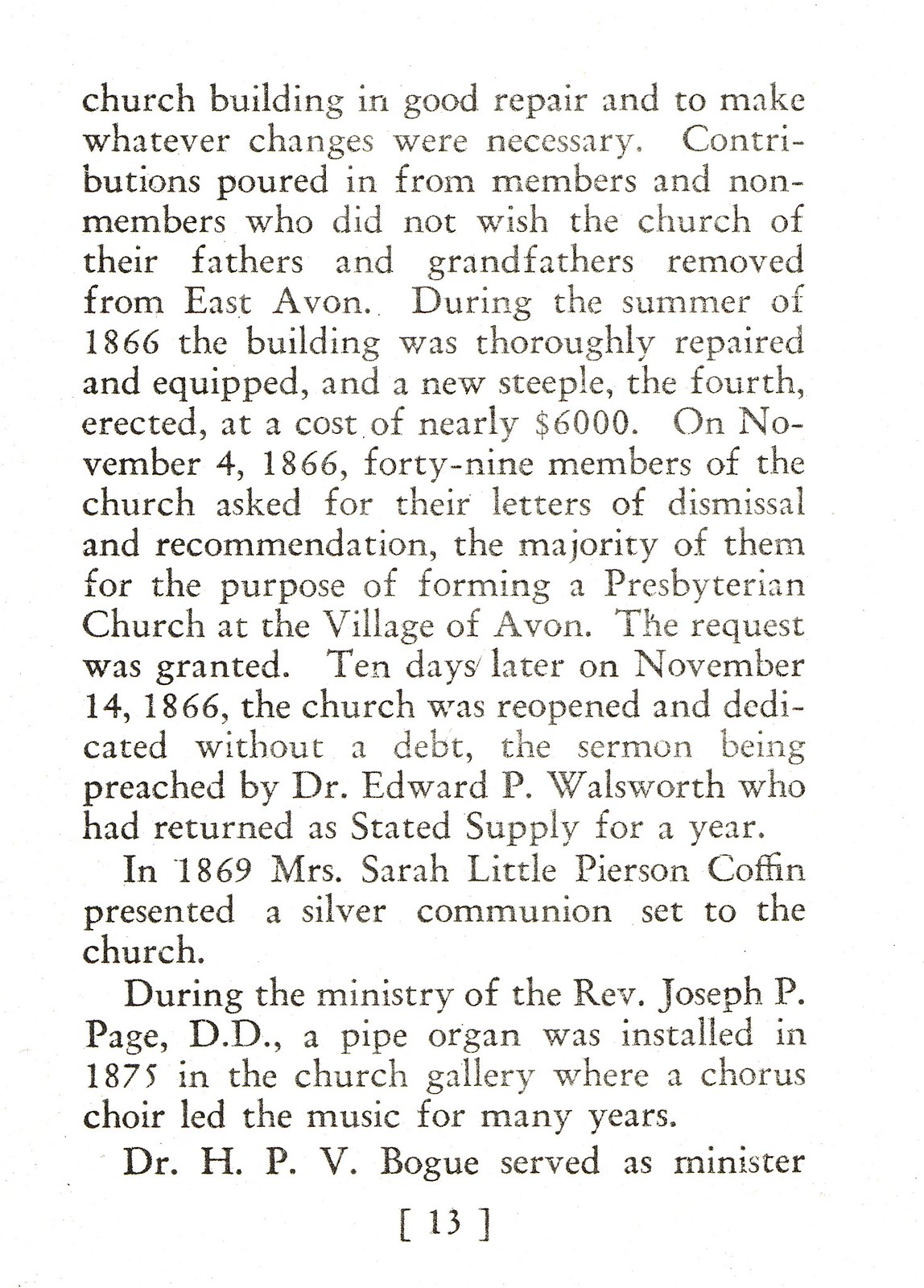The image features black Times New Roman text on a slightly faded white background. The text narrates the history of a church building in East Avon, stating it was in good repair and detailing the necessary changes. It mentions that contributions poured in from both members and non-members who did not wish for the church of their ancestors to be removed from East Avon. During the summer of 1866, the building was thoroughly repaired and equipped with a new steeple, the fourth one, costing nearly $6,000. On November 4th, 1866, 49 members requested letters of dismissal and recommendation to form a Presbyterian church in the village of Avon, which was granted. Subsequently, on November 14th, 1866, the church was reopened and dedicated without debt, marked by a sermon from Dr. Edward P. Walsworth, who returned as a stated supply for a year. In 1869, Mrs. Sarah Little Pearson Coffin gifted a silver communion set to the church. During Reverend Joseph P. Page, D.D.'s ministry, a pipe organ was installed in 1875 in the church gallery, where choirs had led music for many years. Dr. H.P.V. Bogue also served as a minister. At the bottom, the number 13 appears in parentheses.